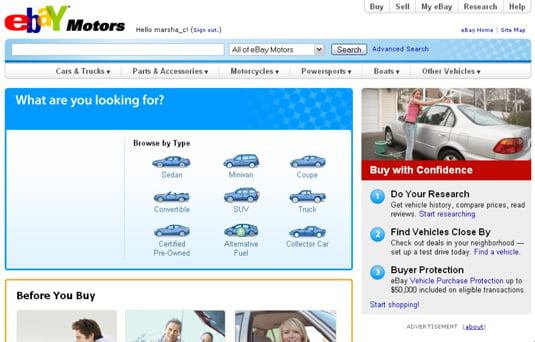The screenshot of the eBay Motors website showcases a detailed and organized interface. At the top left, the "eBay Motors" logo is prominently displayed. "eBay" features an older style with each letter in a different color: E in red, B in blue, A in yellow, and Y in green, followed by "Motors" in black. Adjacent to the logo, the text "HelloMarsha_CF" appears, with a blue "sign out" option beside it.

In the top right corner, there are several navigation buttons labeled "Buy," "Sell," "My eBay," "Research," and "Help." Below these, options for "My eBay Home" and "Site Map" are available. A search bar, designed as a long white rectangle, is located to the left with a drop-down menu set to "All of eBay Motors" and a search button. Nearby, the "Advanced Search" option is highlighted in blue.

Further down, horizontal drop-down menus include categories such as "Cars & Trucks," "Parts & Accessories," "Motorcycles," "Powersports," "Boats," and "Other Vehicles." A blue banner with white text reads, "What are you looking for?" followed by silhouettes of various vehicle types, including sedans, convertibles, SUVs, and trucks—nine in total.

To the right of these silhouettes, an image depicts a young woman washing a gray sedan. She is wearing a pink tank top and blue jeans. Below this image, the text "Buy with Confidence" is visible. Additional sections labeled "Do Your Research," "Find Vehicles Close By," and "Buyer Protection" offer further information with accompanying black text.

At the bottom left, a section titled "Before You Buy" is accompanied by three photographs, each depicting individuals either inside or near vehicles. The overall webpage screenshot features a predominantly white background.